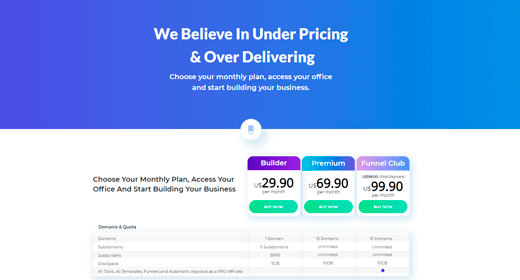This image is a screenshot showcasing various subscription or monthly plan options, though it does not specify the product or service explicitly. 

At the top of the screenshot, there is a prominent thick blue banner with the following text in white: "We believe in underpricing and over-delivering. Choose your monthly plan, access your office, and start building your business." Beneath this banner, there is a small white circle containing a blue, upside-down lock icon, suggesting security or restricted access.

On the left-hand side, the same text from the banner is repeated: "Choose your monthly plan, access your office, and start building your business." 

Below this, three different subscription plans are displayed:

1. **Builder Plan**: 
   - Cost: $29.90 per month
   - Banner Color: Purple
   - Includes an unreadable green button.

2. **Premium Plan**:
   - Cost: $69.90 per month
   - Banner Color: Blue
   - Includes a green button labeled “Buy Now.”

3. **Funnel Club Plan**:
   - Cost: $99.90 per month
   - Banner Color: Not specified
   - Includes a green button labeled “Buy Now.”

Below these options, there is a longer bar that includes the text “Domains and Quote,” followed by a list comprising five lines of information about each of the three plans. However, the text in these lines is light and difficult to read.